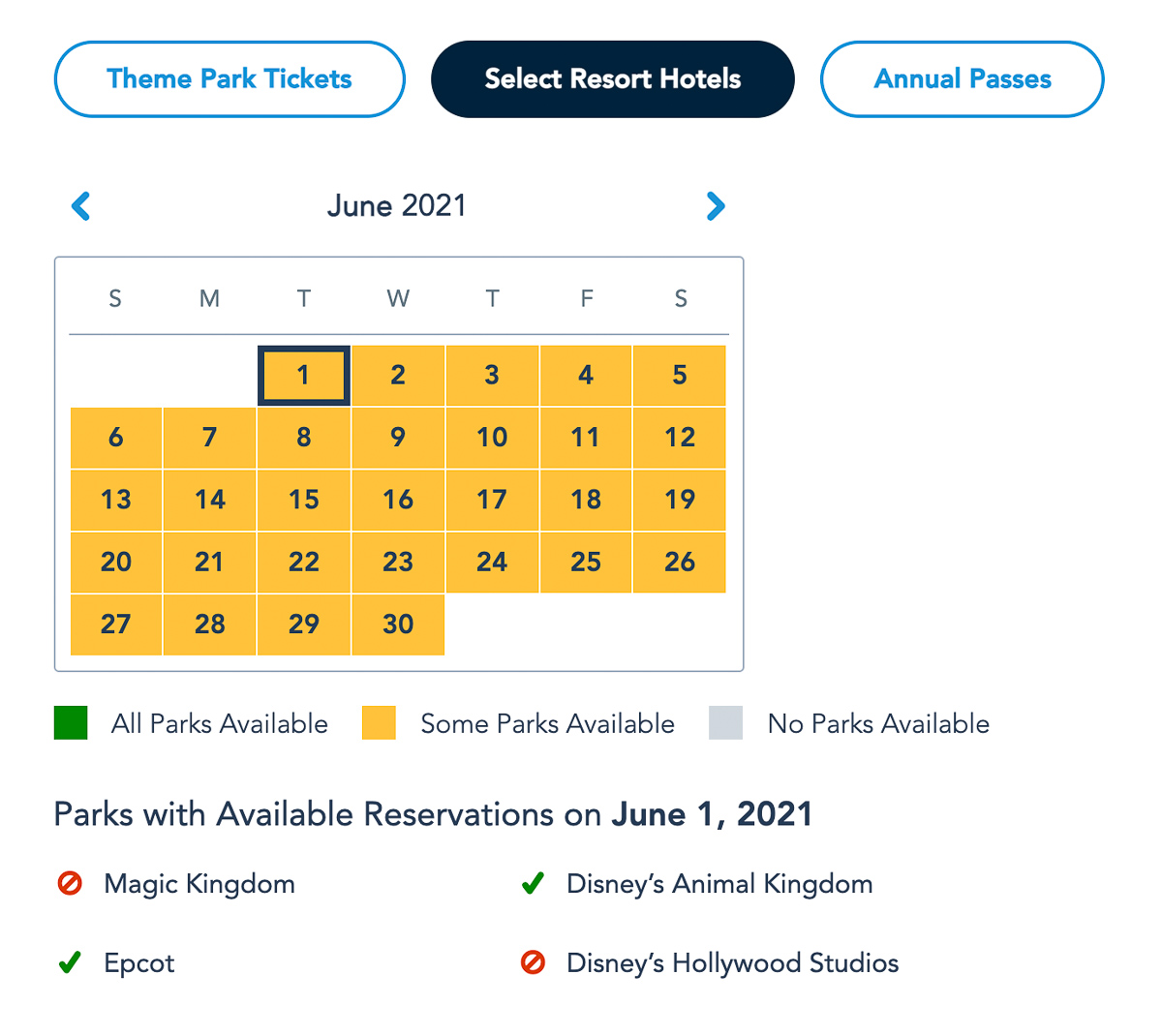A detailed calendar interface for June 2021 displays several interactive elements and information pertaining to park availability. At the top, three options are presented: "Theme Park Tickets" on the left, "Annual Passes" on the right, both encapsulated in a blue oval with a white background and blue text, and "Select Resort Hotels" in the center with a black background and white text.

The calendar itself shows a standard monthly grid starting on Sunday (SMTWTFS) with individual dates numbered 1 to 30. June 1 begins on a Tuesday and the month's last day, June 30, falls on a Wednesday. Each date is highlighted with a yellow background, signifying some form of park availability. The date currently selected is emphasized with a black highlight around the number, positioned on a Tuesday.

To interpret the color codes, a legend is provided below the calendar: a green square signifies "All parks available," a yellow square indicates "Some parks available," and a gray square means "No parks available."

Beneath the legend are details for reservations on June 1, 2021. Reservations are split into two sections: 

- On the left:
  - Magic Kingdom: Unavailable (indicated by a red cancellation icon)
  - Epcot: Available (indicated by a green checkmark)
  
- On the right:
  - Disney's Animal Kingdom: Available (indicated by a green checkmark)
  - Disney's Hollywood Studios: Unavailable (indicated by a red cancellation icon)

The entire layout is displayed on a white background, ensuring clear visibility and contrast for all elements.